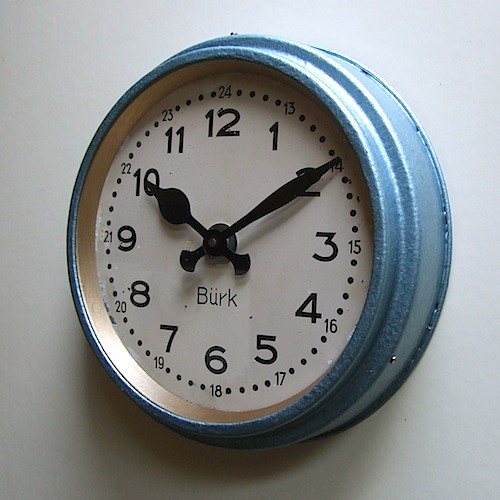This photograph captures a meticulously detailed clock mounted on a pristine white wall. The clock, with its circular design, features a striking blue pearlescent metal outer edge, seamlessly transitioning into a bronze-gold inner rim that contrasts beautifully against the white face. Bold black numerals mark each hour, accompanied by a corresponding 24-hour notation above each number, such as "13" above "1" and "18" above "6". The time displayed is 10 past 10, indicated by the prominent, chunky black minute and hour hands. The design elements of the clock come together to create a timeless yet modern aesthetic.